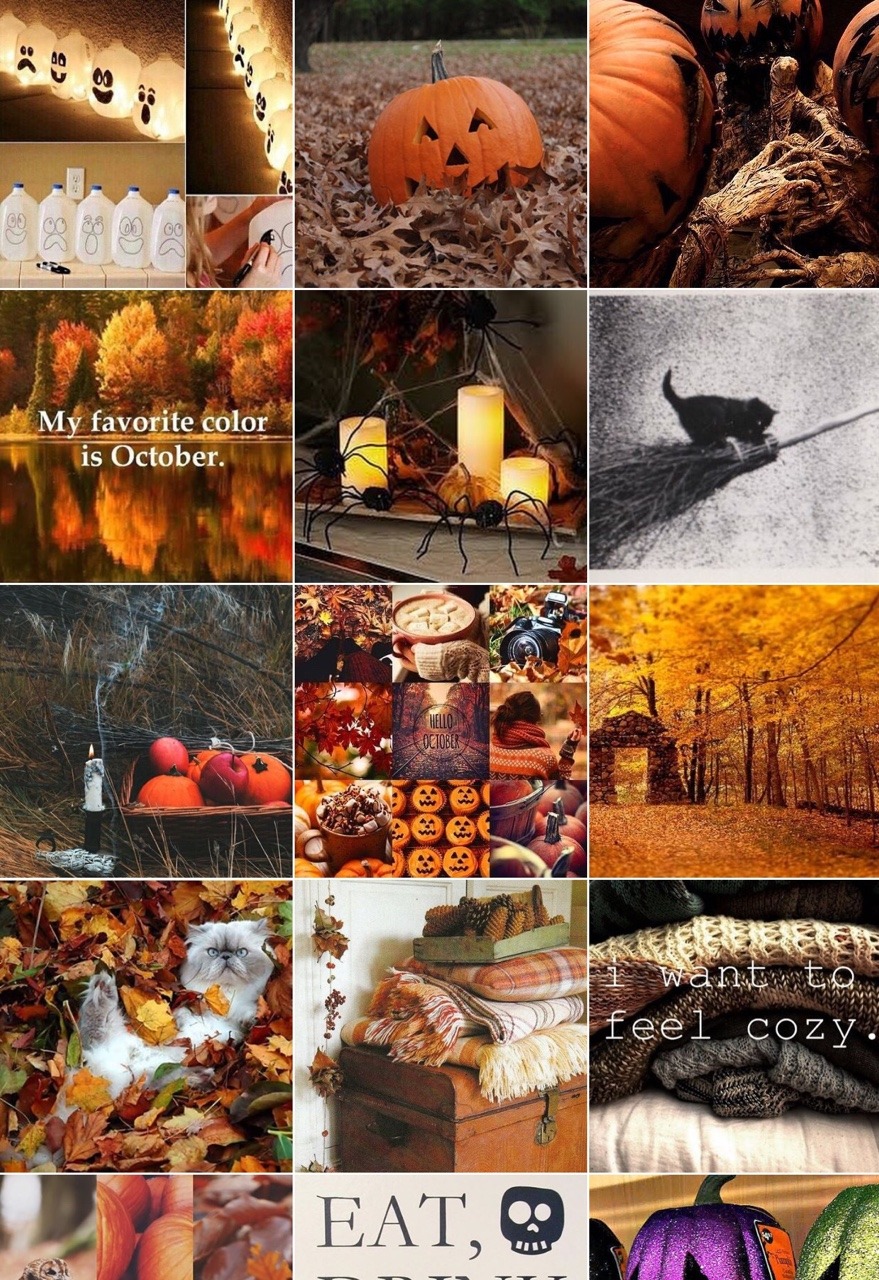This collage features a variety of Halloween and autumn-themed images, organized in a grid with five rows of three columns, though the bottom row has been cropped out.

- The top left image displays a row of milk jugs that have been artistically painted to resemble ghosts, each with a candle flickering inside, creating a spooky yet charming effect.
- To the right of this, there is a photo of a jack-o-lantern nestled within an autumnal pile of leaves, capturing the essence of fall perfectly.
- Below the jack-o-lantern, on the left side, a decorative sign reads, "My favorite color is October," celebrating the season with a playful twist.
- Adjacent to this sign, three candles burn brightly among scattered fake spiders, enhancing the Halloween spooky ambiance.
- To the far right, a whimsical illustration depicts a cat flying on a broomstick, adding a touch of magical mischief.
- Moving down a row to the left, a large container brimming with pumpkins showcases the harvest's bounty.
- Next to that, a mouthwatering display of Halloween-themed desserts, including vibrant orange cookies, tempts with seasonal treats.
- Finally, completing the row, an image captures trees shedding their leaves in a flurry of fall colors, a picturesque representation of the season's transition.

Overall, the collage beautifully encapsulates the spirit of October and Halloween through an array of visually engaging and thematic photos.